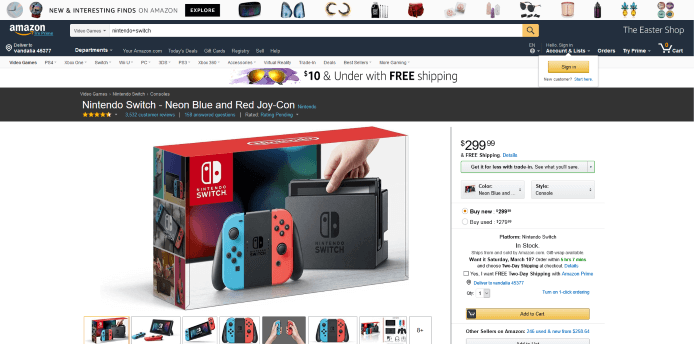This is a detailed caption for the image originally described:

The image is a horizontal rectangle taken from an Amazon webpage. At the top of the page, several icons are aligned along the top border from left to right. Following the first two icons, the text "NEW AND INTERESTING FINDS" is displayed in bold, black, all-caps font, followed by "on Amazon" in a regular font.

Below this section, a black rectangular banner covers the width of the image. In the upper left corner of this banner, "amazon" is written in white, lowercase letters next to the iconic Amazon logo, featuring a yellow arrow pointing from "a" to "z". Additionally, a bold white address, not the user's but a generic one, appears under this logo. The only readable menu item in bold white font is labeled "DEPARTMENTS." On the opposite side (top right), "The Easter Shop" is displayed in white font on this same dark area, potentially navy blue. Below this is an icon of a shopping cart accompanied by the word "Cart."

The following section of the image is white and extends from left to right, showcasing various unreadable menu items. In the center of this section, there is an image of sunglasses with orange lenses against a purple backdrop, along with the price "$10" in bold black font. Below the price, the text "with FREE shipping" is displayed, emphasizing "FREE" in all capitalized, bold lettering.

Just below, there is another almost black rectangular area extending from left to right. In this section, "Nintendo Switch, Neon Blue and Red, Joy-Con" is written in bold white font, referring to the controllers. Below, four and a half yellow stars are depicted, indicating a rating, with some unreadable small blue text (possibly turquoise).

Underneath this, a box appears at a diagonal angle (catty-corner). The right side points toward the upper right corner, and the left side points to the lower left. The top of the box is red with white lettering. The front features a red area with white text saying "Nintendo Switch" in all-capital white letters, with "Switch" being more prominent. It also includes an icon of the controllers in red and white.

Further in this section, there is a visual of the actual Nintendo Switch controllers, showcasing a blue left side, a black middle, and a red right side, all connected. A hand extends from the upper right corner, pulling an item from the black box labeled "Nintendo Switch". Below are smaller images of the device.

To the right of these visuals, the price "$299.99" is displayed in black font, followed by "FREE" in all caps, and "shipping" in regular font. Additionally, "details" is written in turquoise font beside them, hinting at more information available.

At the bottom of the image, there is a yellow rectangular button with the words "Add to Cart" in black.